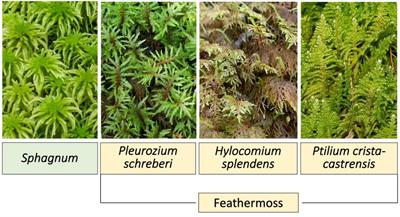The image is a detailed chart of four different types of mosses, each displayed within a vertical rectangular segment. On the left side, the first rectangle features a green plant with spidery leaves, labeled "Sphagnum" in a green box with black text. Adjacent to this are three additional rectangles grouped together with a bracket and labeled individually. The first of these shows a blue-tinged, spidery green plant labeled "Plerosium shrubbery" in a tan box with black text. The second rectangle displays a mossy-looking plant that is a mix of dark brown and pale green, labeled "Hylacomium splendens" in a pale yellow box. The final rectangle in this group depicts a pale yellow and green spindly plant, labeled "Tillium christicostrensis" in a yellow box. Beneath these three grouped images, there is a pale yellow box with black text that reads "Feather moss." The overall color palette of the photo predominantly involves shades of green, with some brown and yellow variations.